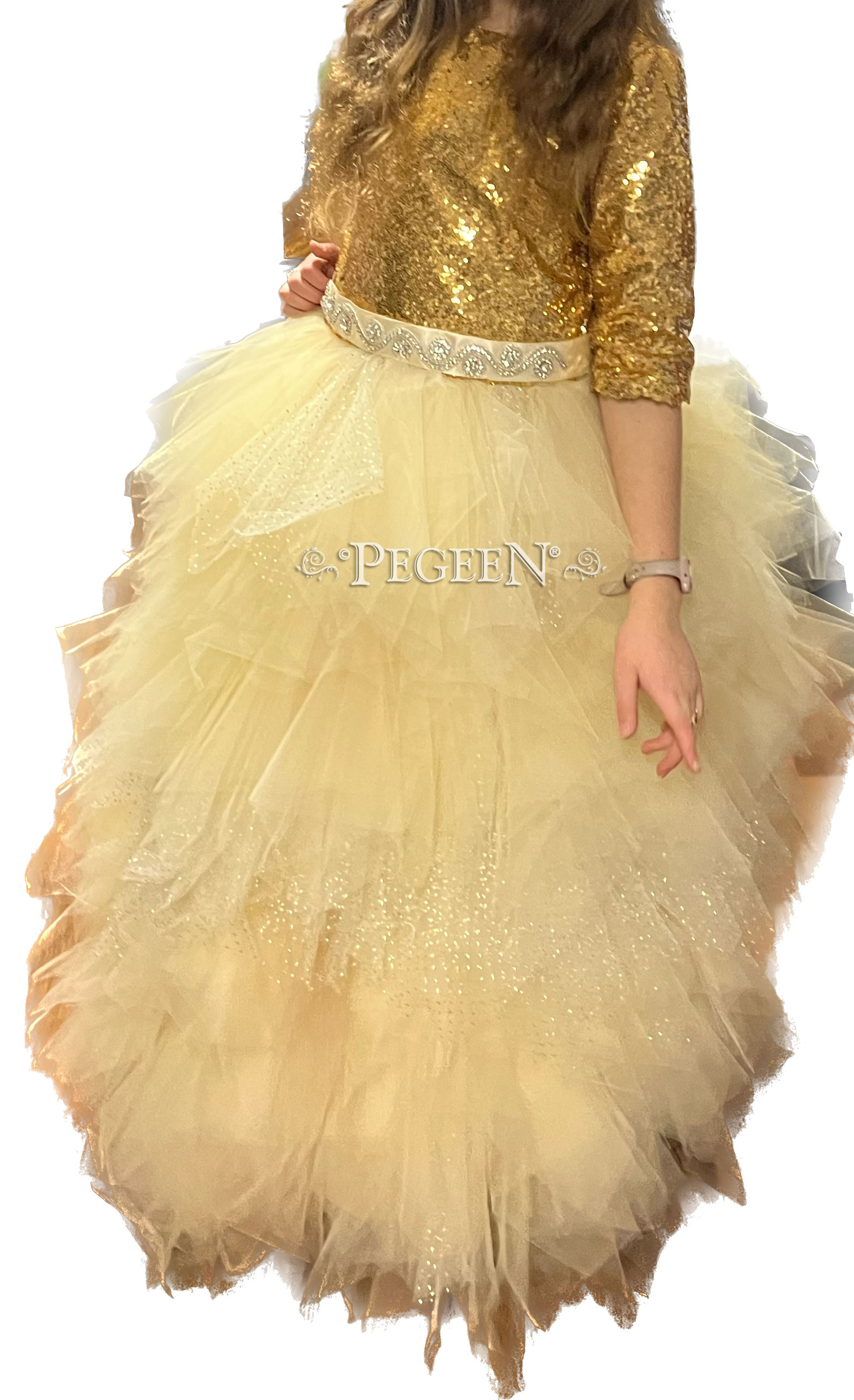In this promotional image with a PEGEN watermark at the center, a woman's glamorous outfit is showcased from the neck down. The centerpiece of the ensemble is a voluminous, puffy skirt made of a silky, layered material in varying shades of light tan, darker brown, and dark gray. The skirt flows gracefully to the floor, completely covering her feet. Her top is a striking gold lamé or sequined shirt with sleeves pushed up to just below the elbow. Accentuating the waist is a stylish belt or waistband in a lighter gold tone, adorned with intricate silver beading and white jewel decorations. The overall look is one of opulent elegance, highlighted by the shimmering textures and detailed embellishments.